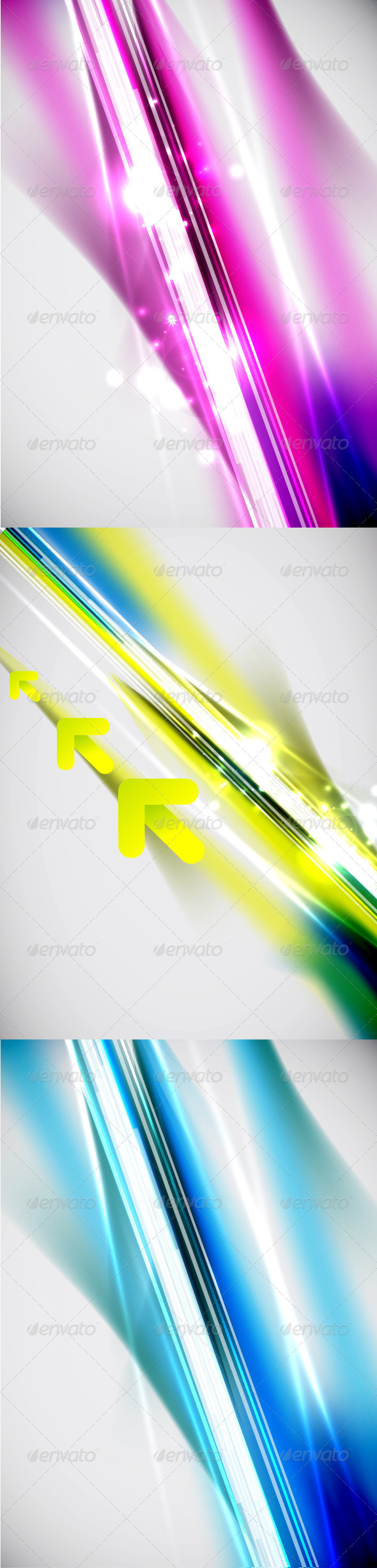The image features three vertically stacked picture cards against a white brick wall. Each card showcases a distinct yet similar striped, glittery pattern, appearing as if paint is being poured diagonally with a dynamic sense of motion. The top card displays magenta, pink, and white streaks that shine and sparkle. The middle card features yellow, blue, and cyan streaks, with three smaller arrows pointing upward from the lower portion of the card. The bottom card presents dark blue, light blue, and white streaks. The glittery, computer-generated design of each section gives the impression of internal illumination, adding depth and vibrancy to the colorful artwork that occupies most of the frame.